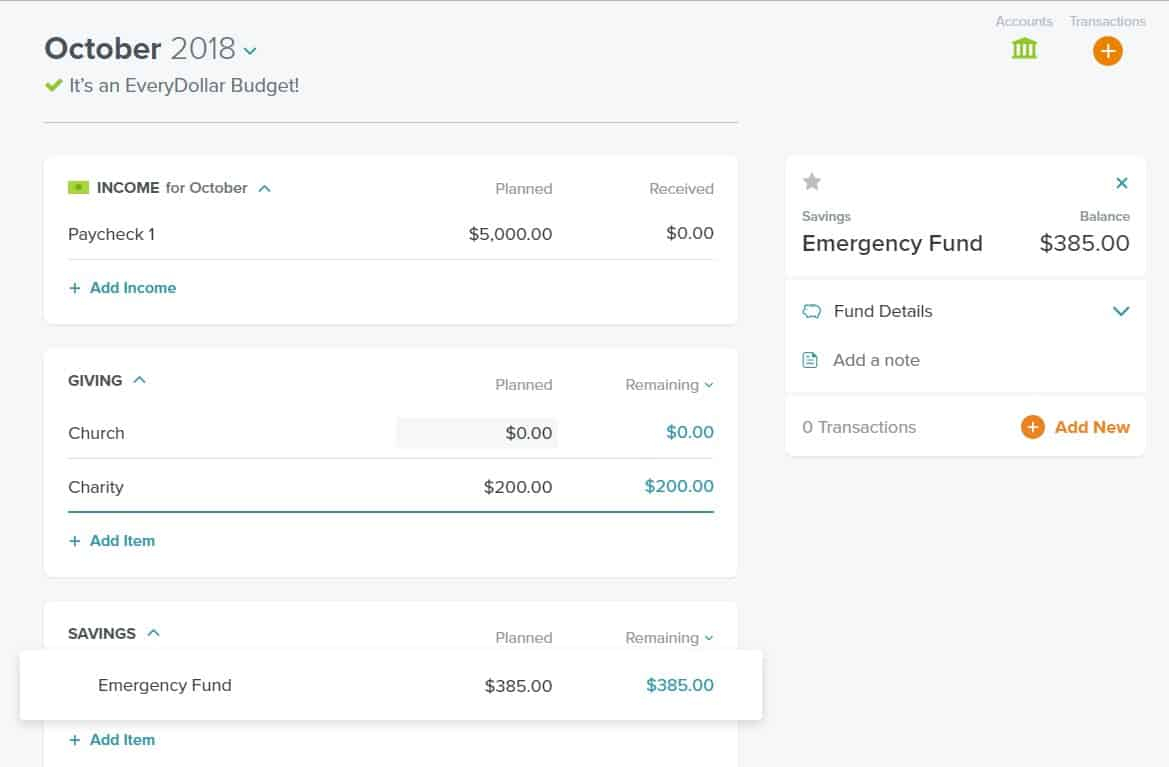This image depicts a budgeting interface for October 2018, characterized by an "EveryDollar" budget layout. Prominently displayed is a green checkmark indicating completion or accuracy. The "Income for October" section lists a planned paycheck of $5,000. 

In the "Giving" category, two items are shown: "Church" with no allocated amount and "Charity" with a planned donation of $200. 

The "Savings" category features an "Emergency Fund" line item, which highlights an emergency fund savings of $385. This amount appears twice: once under the planned savings area and again in a balance section to the right, both marked in blue. Additionally, the interface offers options to "Add a Note" or "Add New," the latter represented by an orange button with a cross. 

Overall, the user appears to be reviewing transactions within their accounts.